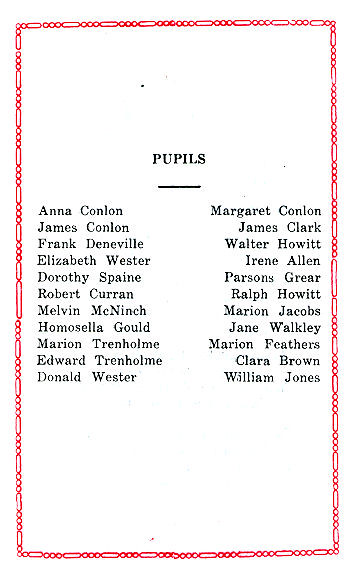The image appears to be a page from a pamphlet, possibly from a conference or church handout. It features a distinctive red border resembling a rope with circular designs. The background is white with black text. At the top center, the word "Pupils" is prominently displayed. Below this heading, there is a horizontal line followed by a two-column list of names. The left column includes Anna Conlon, James Conlon, Frank D. Neville, Elizabeth Wester, Dorothy Spain, Robert Kirk Curran, Melvin McNinch, Homosella Gould, Marion Trenholm, Edward Trenholm, and Donald Wester. The right column lists Margaret Conlon, James Clark, Walter Howitt, Irene Allen, Parsons Greer, Ralph Howitt, Marion Jacobs, Jane Walkley, Marion Feathers, Clara Brown, and William Jones. The layout features substantial white space below the names, contributing to a clean and organized appearance.